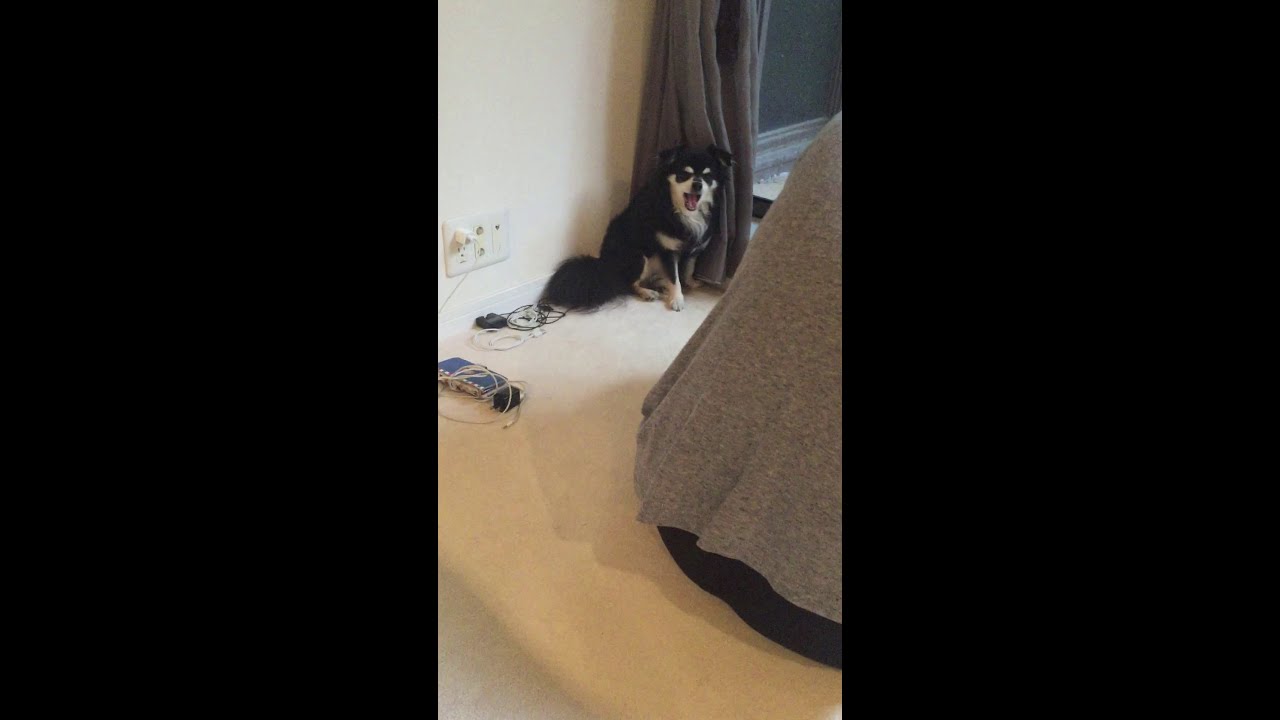In the image, a small black and white dog with attentive, slightly upright ears is sitting on a very light yellow, almost cream-colored carpet. The dog has distinctive yellow markings on its face, chest, and paws. Its mouth is open, revealing a hint of redness inside, and it has black patches over its eyes. The dog is seated directly against a white wall, beside which a gray curtain hangs from the ceiling, partially obscuring a window with a visible bottom black frame. The wall features a power outlet on the left with a white cable plugged into it, trailing towards the bottom left. To the right of the image, a person sits on a bed, their back facing the camera. They are dressed in a gray shirt and black pants. The person's presence and the bed cast subtle shadows on the carpet. The overall setting suggests a cozy, domestic environment with nuanced details such as electrical cords on the floor that add to the scene’s lived-in feel.